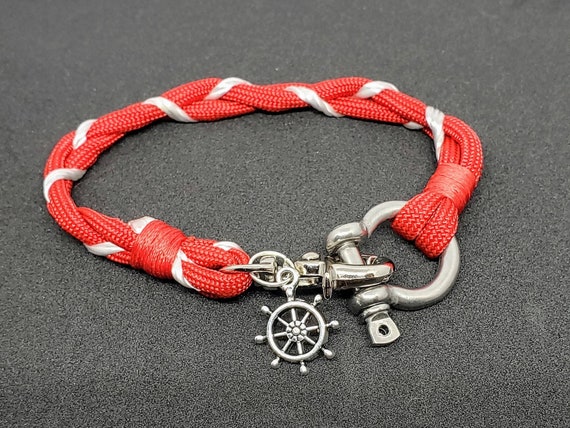This image features a striking bracelet displayed on a dark gray, slightly rough surface. The bracelet itself is crafted from thin, red rope interwoven with white strands, giving it a twisted and braided appearance. This elegant design forms a circle that could comfortably fit around a wrist. Central to the bracelet is an intricate silver clasp, comprised of two main loops: one fully enclosed and another semicircular loop secured by a pin. The clasp is both functional and ornamental, featuring a small, vintage charm hanging from it—a detailed ship's wheel reminiscent of those from old-time pirate ships, complete with several spokes extending outward. The overall presentation highlights the bracelet's nautical theme and meticulous craftsmanship.